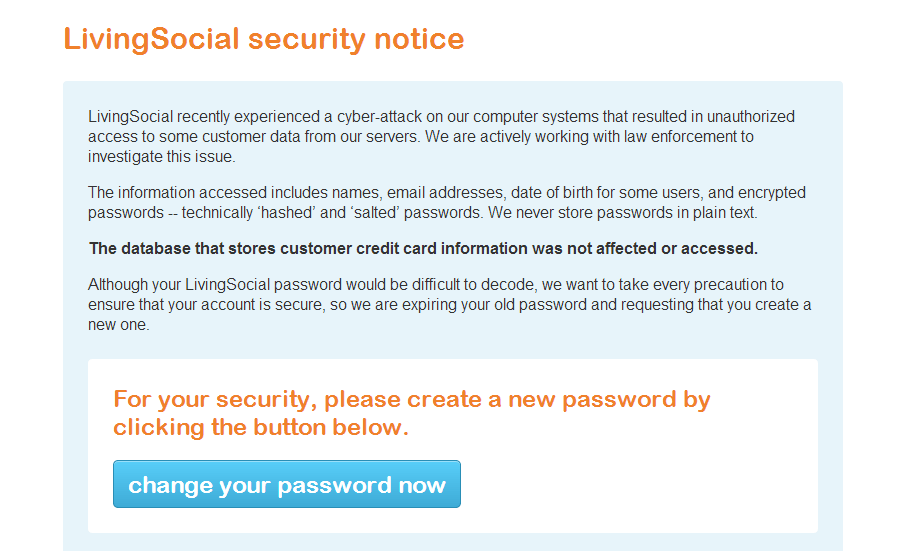A horizontally rectangular image is framed with a white border. At the top left corner of the border, the words "LivingSocial" appear in orange, written without space between them. Below the border is the header "Security Notice," followed by a light blue, horizontally rectangular box containing important information.

The text inside the light blue box explains that LivingSocial recently experienced a cyber attack, resulting in unauthorized access to some customer data stored on their servers. The company is actively collaborating with law enforcement agencies to investigate the issue. Compromised information includes customer names, email addresses, dates of birth for some users, and encrypted (hashed) passwords. It is emphasized that LivingSocial does not store passwords in plain text.

A bold line states: "The database that stores customer credit card information was not affected or accessed."

The following unbolded text assures users that although their passwords would be difficult to decode, LivingSocial is expiring the old passwords as a precautionary measure. Users are requested to create new passwords to ensure account security.

Beneath this, within the light blue background, there is a white, horizontally rectangular box with a message in orange: "For your security, please create a new password by clicking the button below."

At the bottom, a light blue button with the white text "Change Your Password Now" is prominently displayed, inviting users to take immediate action.